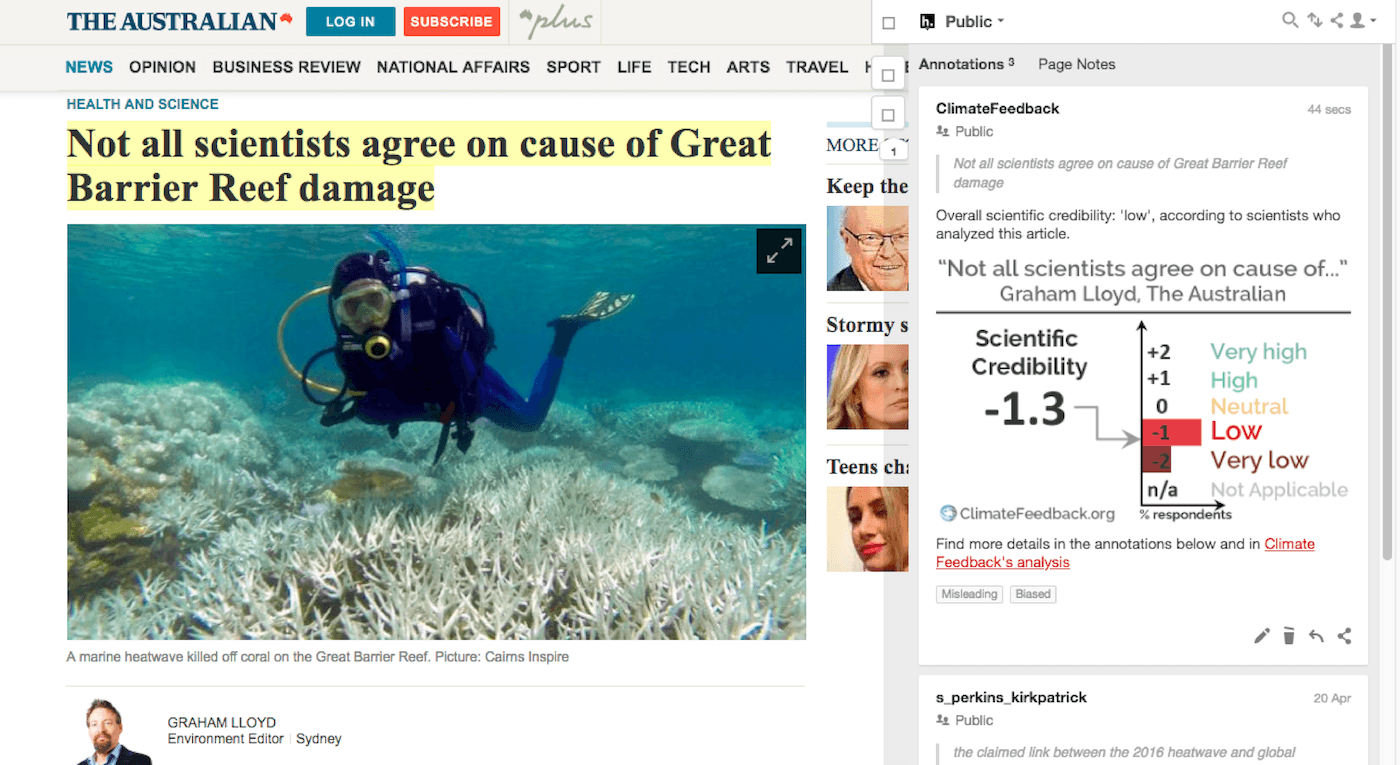The image is a screenshot of an article featured on The Australian. In the upper left corner, the website's branding is displayed, accompanied by a login button and a subscribe option. Below, various navigation tabs are visible, including News, Opinion, Business Review, National Affairs, Sport, Life, Tech, Arts, and Travel. The article falls under the 'Health and Science' category and is titled, "Not all scientists agree on cause of Great Barrier Reef damage."

The main visual in the article shows a scuba diver underwater, navigating near a bed of bleached coral reefs that are predominantly white and spiky, indicative of significant environmental stress. The image caption reads, "A marine heat wave killed off coral on the Great Barrier Reef." This photograph is credited to Calm and Spire.

In the bottom left corner of the article, the byline indicates the piece is written by Graham Lloyd, the Environment Editor based in Sydney, whose photograph — a professional-looking man dressed in a suit gazing towards the camera — is also displayed. To the right side of the screenshot, there is a section for public annotations and page notes, inviting reader interaction and commentary.